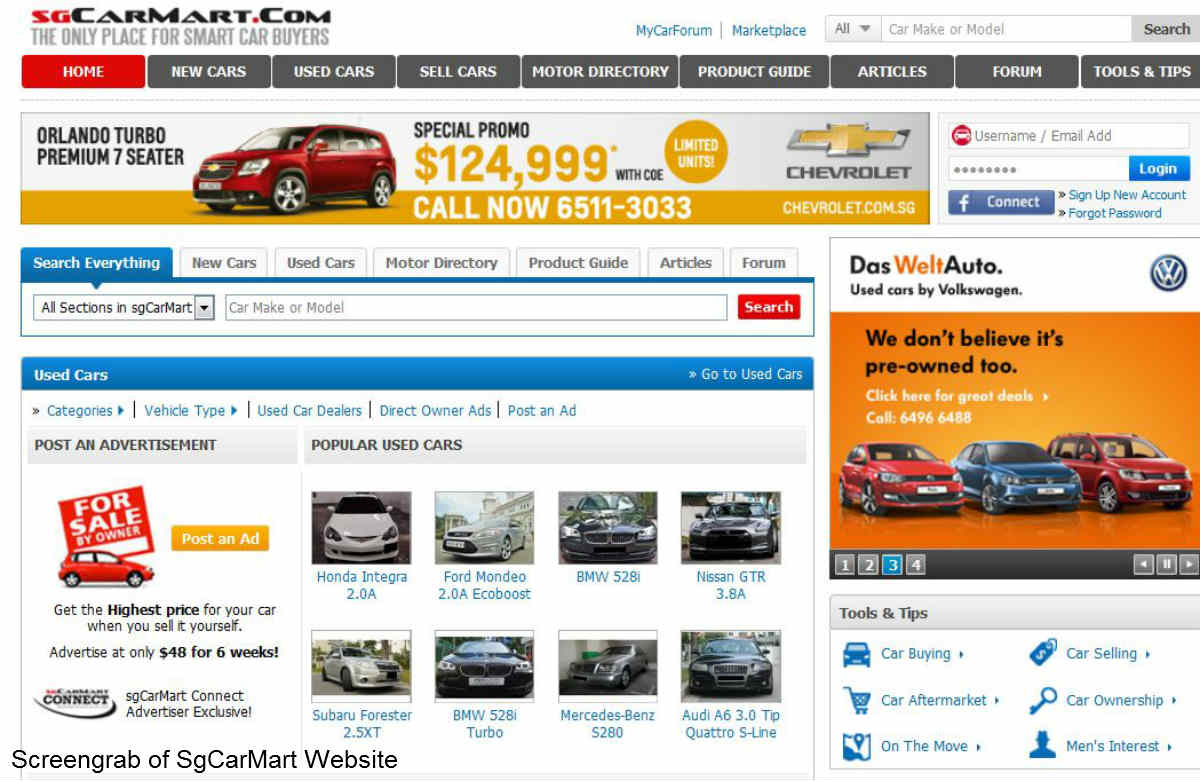A screenshot of an automotive car selling website, CarMart.com, features its logo with "SG" in red and the tagline "The only place for smart car buyers" prominently displayed in the upper left-hand corner. The top navigation bar includes clickable sections for "My Car Forum" and "Marketplace" on the right, along with a comprehensive search function where users can filter by car make or model.

The main navigation menu highlights options such as "Home," "New Car," "Used Car," "Sell Cars," "Motor Directory," "Project Guide," "Articles," "Forum," and "Tools & Tips," with "Home" currently highlighted in red, indicating the user's current page.

Below the navigation bar, a prominent ad showcases the "Orlando Turbo Premium 7 Seater" featuring a Chevrolet vehicle offered at a special promotional price of $124,999 with a Certificate of Entitlement (COE). Limited units are available, and interested buyers are encouraged to call 6511-3033. The ad also includes the Chevrolet logo and the website chevrolet.com.sg.

On the right-hand side of the page, there are login options and a "Facebook Connect" button to facilitate account access.

Further down, users can search for various categories: "New Cars," "Used Cars," "Motor Directory," "Project Guide," "Articles," and "Forums." The site also provides options to explore used cars by categories, type of vehicles, used car dealers, direct owner ads, or even posting an ad.

An enticing advertisement encourages users to "Get the highest price for your car when you sell it yourself," with a promotional offer to advertise for $48 for six weeks. Popular used cars listed include the Hyundai Integra, Ford Mondeo, BMW 528i, Nissan GTR, Subaru Forester, BMW 528i Turbo, Mercedes-Benz 328, and Audi A6 Quattro S-Line.